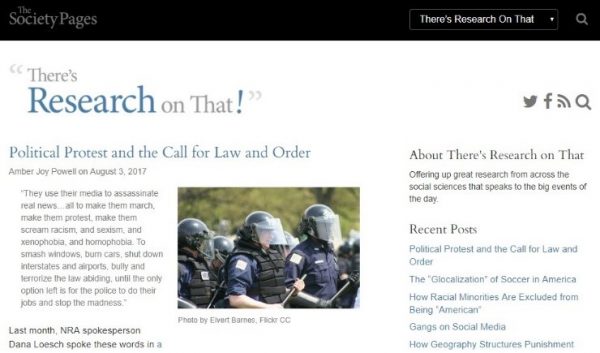The image captures a webpage titled "There's Research On That!" prominently displayed at the top left of a white section. Above this, a heading titled "The Society Pages" is presented on a black background, with a search option located to its right for easy information retrieval. The page's tagline reads: "Offering up great research from across the social sciences that speaks to the big events of the day." The site also features links to various social media platforms, including Twitter (using the old logo before rebranding to X) and Facebook. The front page on "The Society Pages" showcases the most recent post, titled "Political Protest and the Call for Law and Order," written by Amber J. Powell on August 3, 2017. To the right are additional recent posts, including topics such as "The Globalization of Soccer in America," "Gangs and Social Media," "Hydrography Structures," "Punishment," and more, all listed in a sidebar.